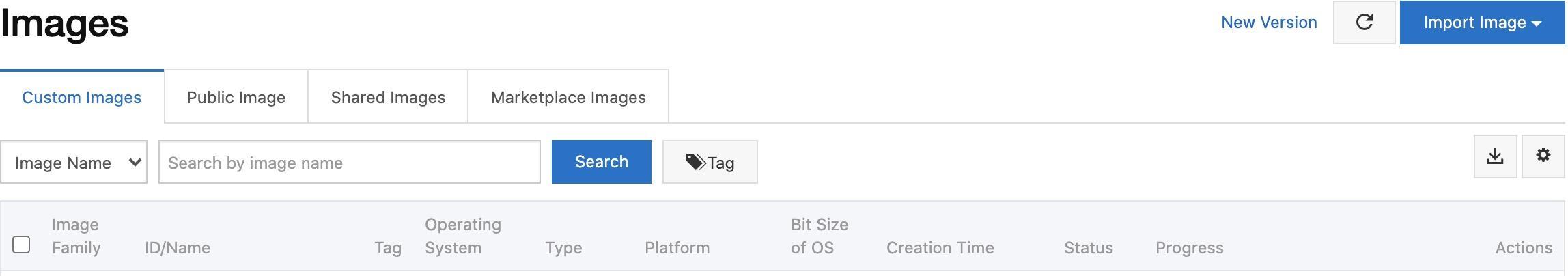**Detailed Caption:**

A user is currently navigating the "Custom Images" section of an image management platform. At the top of the interface, the title "Images" is prominently displayed in black. To its right are three action buttons: "New Version," "Refresh," and a blue "Import Image" button with a dropdown menu.

Below this, the section for custom images is clearly marked with a blue underline and header text that reads "Custom Images" in blue. Directly underneath, there is a field labeled "Image Name" accompanied by a dropdown box where users can search for images by name. To the right of this field is a blue "Search" button, followed by a "Tag" button. Finally, to the far right, there are two icons: a gear symbol for settings and a download button.

The main area, which is a light gray box, is currently empty as there are no customized images listed. This area includes a detailed table with columns labeled: Image Family, ID Name, Tag, Operating System, Type, Platform, Bit Size, Creation Time, Status, Progress, and Actions. Despite the blank state, this structured overview implies where the data would appear and how it would be organized.